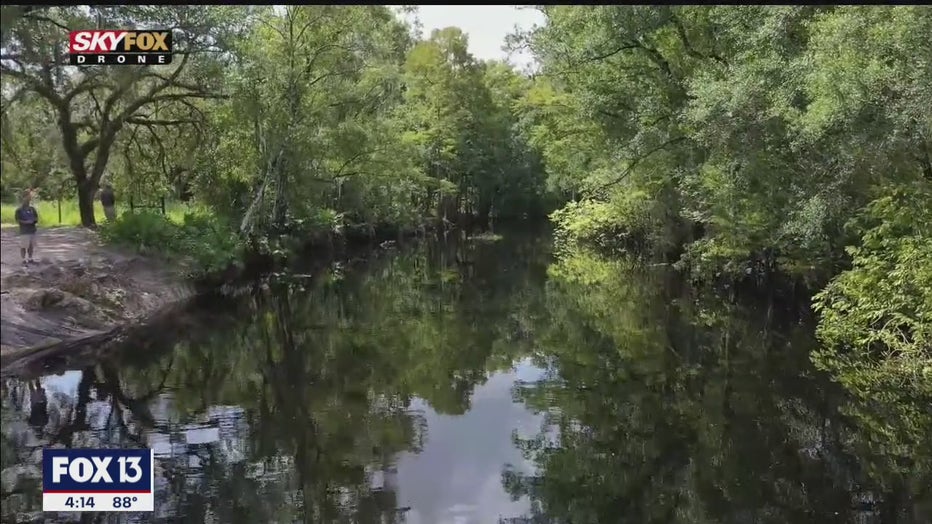A captivating aerial photograph taken from a Sky Fox Drone for Fox 13 shows a tranquil river, possibly a creek, flowing toward the camera. The scene is enveloped in lush greenery, with trees densely lining both sides and slightly leaning over the river, creating a picturesque natural canopy. The remarkably still water mirrors the surrounding foliage and sky with precise clarity, adding a serene, almost surreal quality to the image. In the bottom left corner, a blue and white box with "FOX 13" in white text and the time "414" and temperature "88 degrees" in black beneath it can be seen. Additionally, the upper left corner prominently features red, black, and gold boxes with "SKY FOX" and "DRONE" inscribed within them. In the foreground to the left, a man stands by the minimal shoreline, gazing toward the water, while another man is visible in the background beside a large tree. The scene exudes calmness, with the subtle ripples in the water suggesting a recent disturbance, possibly by someone standing on the shore.